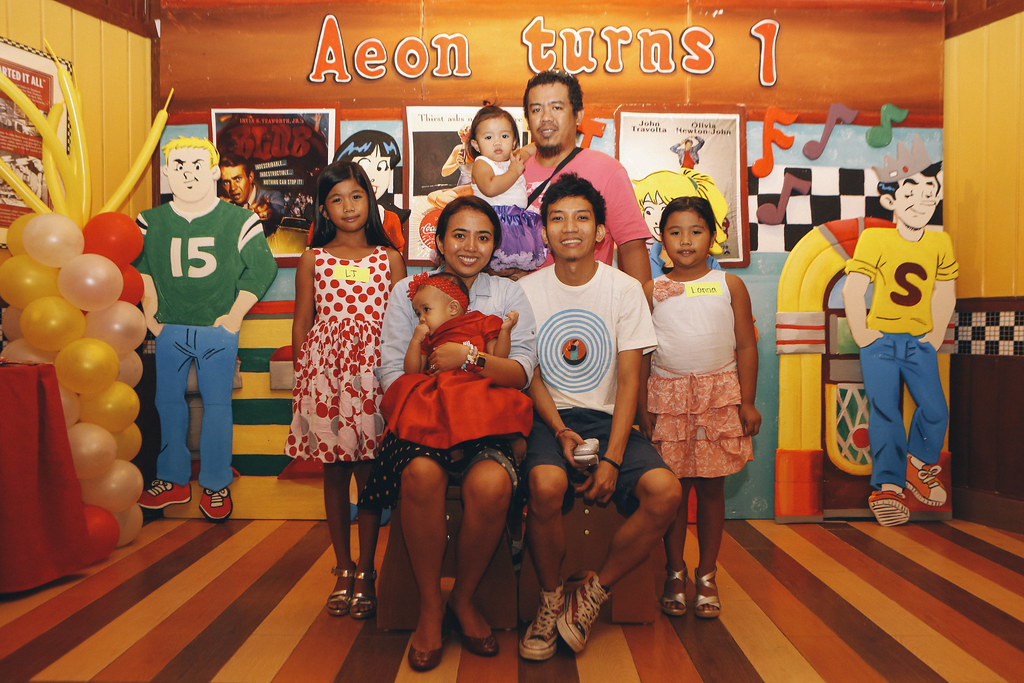This photograph captures a jubilant family gathering for Aeon's first birthday celebration, set against a lively backdrop inspired by Archie Comics. The venue is adorned with various colorful decorations, including movie posters, cardboard cutouts of iconic Archie characters like Jughead beside a jukebox, and a statue of balloons on the left. The whole setting features vibrant hues of orange, brown, and yellow, giving it a nostalgic, 50's diner ambiance. Above the scene, a sign in an Archie-style font proudly declares "Aeon Turns One."

In the background, a man in his 30s, sporting a goatee and a pink shirt, stands holding a young girl dressed in a purple and white outfit. Below him, a row of family members is seated and standing. The first is a young girl about 10 or 11 years old, dressed in a white and red polka-dotted dress and long black hair, with the initials "LT" on her dress. Next to her stands another young girl in a white tank top and pink skirt, adorned with a sticker that reads "Lana."

Seated in front, a woman in her 20s, wearing a blue button-up shirt, cradles baby Aeon in an elegant red dress, suggesting that Aeon is the birthday celebrant. Beside the woman, a young man, also in his 20s, with a goatee and wearing a white t-shirt with a blue circle design, smiles warmly. The floor beneath them appears to be multi-colored wood or tile, adding to the cheerful and festive atmosphere of this family photo.